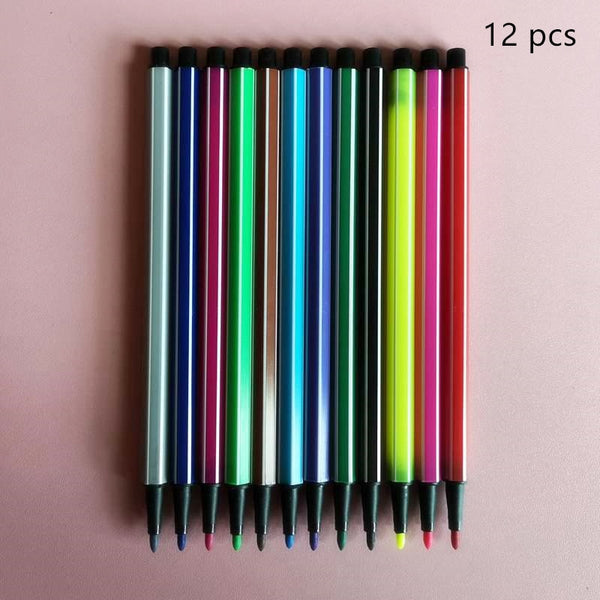This image showcases a set of 12 thin, uncapped markers arranged neatly from right to left on a pink background. The order of the colors is as follows: red, pink, neon yellow, black, dark green, dark blue, light blue, brown, light green, pink, purple, and gray (possibly silver). Each marker features a striped design, with white lines running along the barrel that matches the marker's color. In the upper right-hand corner of the image, black text abbreviates "12 pieces" as "12 PZS". The markers are all uniformly aligned, appearing either in a holder or laid out carefully to display the vibrant array of colors.